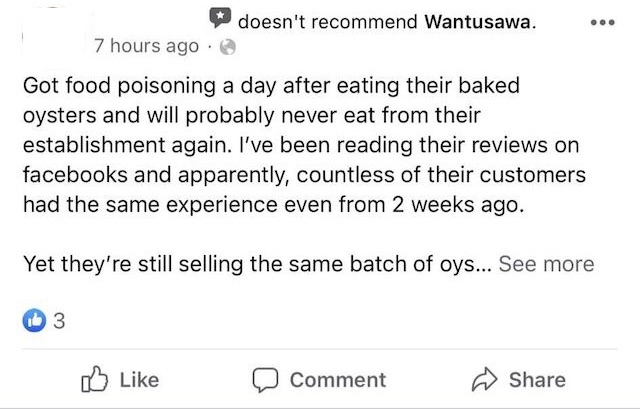### Descriptive Caption:

In this image, we see a screenshot against a solid white background. At the top, there is a black message box with a white star icon on the right side, followed by an ellipsis (three dots) to the far right. Below this, the timestamp "Seven hours ago" is displayed in light gray text.

Underneath the timestamp, in bold black text, is a post that reads:

"Got food poisoning a day after eating their baked oysters and will probably never eat from their establishment again. I’ve been reading their reviews on Facebook and apparently countless of their customers had the same experience even from two weeks ago. Yet they're still selling the same batch of oysters."

At the bottom of the post, there is a "See More" link in gray text, indicating truncation. Below this, the post has received three likes, which is shown by the number on the "like" button at the lower left corner. From left to right, the interactive buttons read: Like, Comment, and Share.